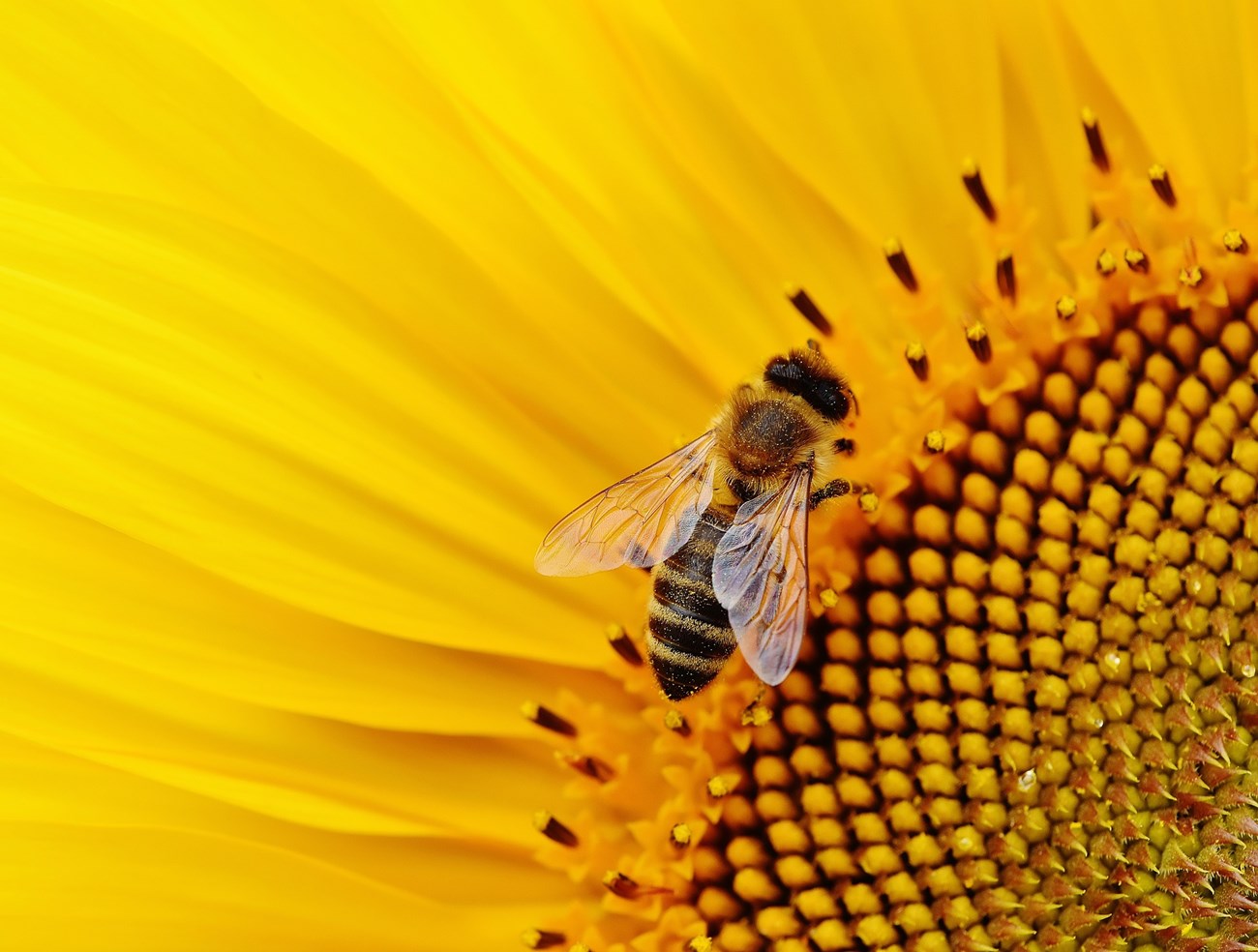In a vivid close-up, a bee is meticulously gathering pollen from a vibrant flower. The frame centers on the bee, whose distinct yellow and black stripes stand out against the intricate details of the flower. The bee's transparent wings are clearly visible, poised delicately as it engages in its task. In the bottom right corner, there's a dense cluster of pollen granules, displaying a varied texture with lighter pieces interspersed among darker fragments. Encircling this corner is a semi-ring of what appears to be the stamen, adding a deeper hue to the scene. Radiating outwards from this point are bright yellow petals, stretching towards the left side and top of the image, creating a bold contrast with the darker pollen. The bee's dark eyes, with a hint of yellow, are focused, and one of its legs is visibly interacting with the pollen, emphasizing the dynamic interaction between the insect and the flower. This close-up captures the intricate details and colors involved in this small yet vital act of nature.